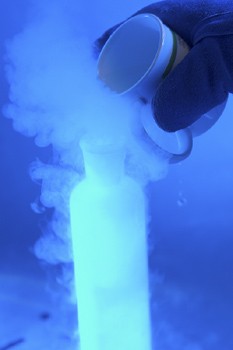In the center of this vertical photograph, a thickly padded, dark blue, or black insulated glove holds a white or bluish-white coffee mug, tilted as it pours into a tall, bluish-white bottle standing upright. The entire scene is bathed in a teal-shaded blue background, creating a blurry and foggy atmosphere. Surrounding the top of the bottle and the area behind the mug is a cloud of light blue fog, likely resulting from the liquid—possibly liquid nitrogen or another chemical—being poured into the bottle, which appears to be glowing with a light blue hue. The interaction between the liquid and the contents of the bottle creates a striking visual effect, with the cloudy gas emanating from the bottle, further adding to the mysterious and scientific ambiance of the image.